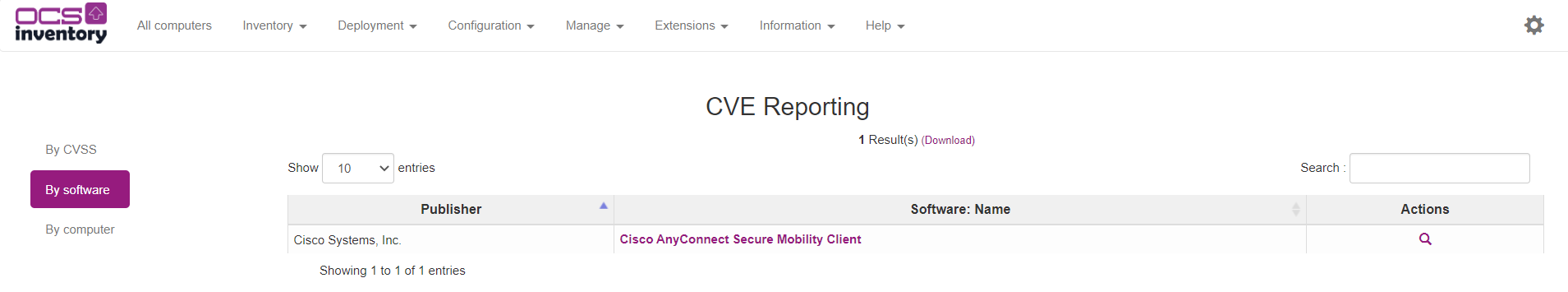This is a cleaned-up and detailed version of the caption:

---

The image is a screenshot of an OCS Inventory web page. The header features the text "OCS" prominently in purple within a purple box that includes an up-arrow, followed by the word "Inventory" in bold black letters. Below the header, the navigation menu is displayed with options in black text on a white background: "All Computers," "Inventory," "Deployment," "Configuration," "Manage," "Extensions," "Information," and "Help," each accompanied by a pull-down menu.

The main section of the page is titled "CVE Reporting" and shows one result with a prominent purple download button. The interface offers an option to display 10 entries at a time, with a search bar situated on the far right. 

The table below lists entries such as "Publisher," with one entry from "Cisco Systems Inc." displayed. The software name "Cisco AnyConnect Secure Mobility Client" is also shown alongside actions for the listed software. There is another search bar aligned to the right for easy filtering.

Additionally, there are filter options including "By CVSS" and "By Software," both enclosed within a purple box with white lettering. Further down, there is an option labeled "By Computer."

---